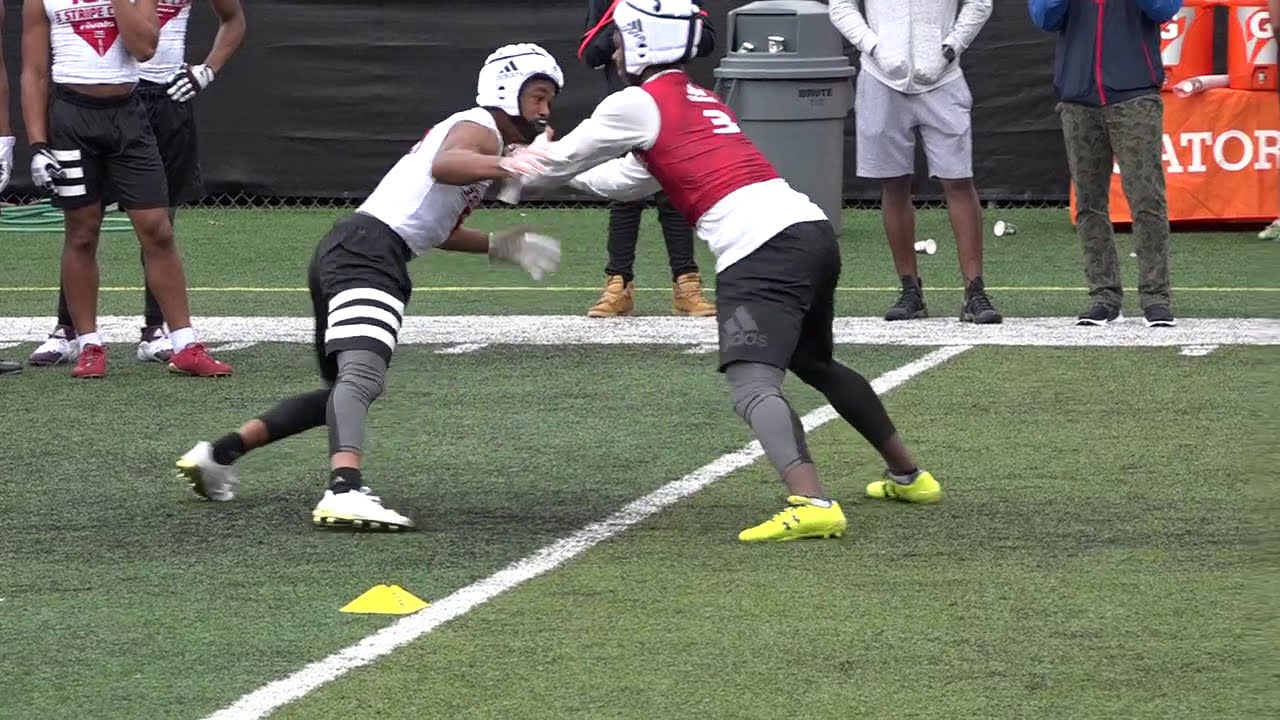In this photograph, two dark-skinned athletes, possibly rugby players, are engaged in a practice session on a grass field marked with white lines. The athlete on the left is dressed in white cleats, black athletic pants, a sleeveless white jersey, and a white helmet, complemented by white goalie gloves. In contrast, the athlete on the right has neon yellow cleats, black and gray athletic shorts, black and gray tights, and a white long-sleeve shirt covered by a red sports vest displaying the number three. Both players are wearing white helmets and appear to be pushing against each other, possibly practicing defensive techniques. In the background, several onlookers can be seen from the torso down, some dressed in regular attire and others in white shirts and black athletic shorts, indicative of fellow players observing the action.